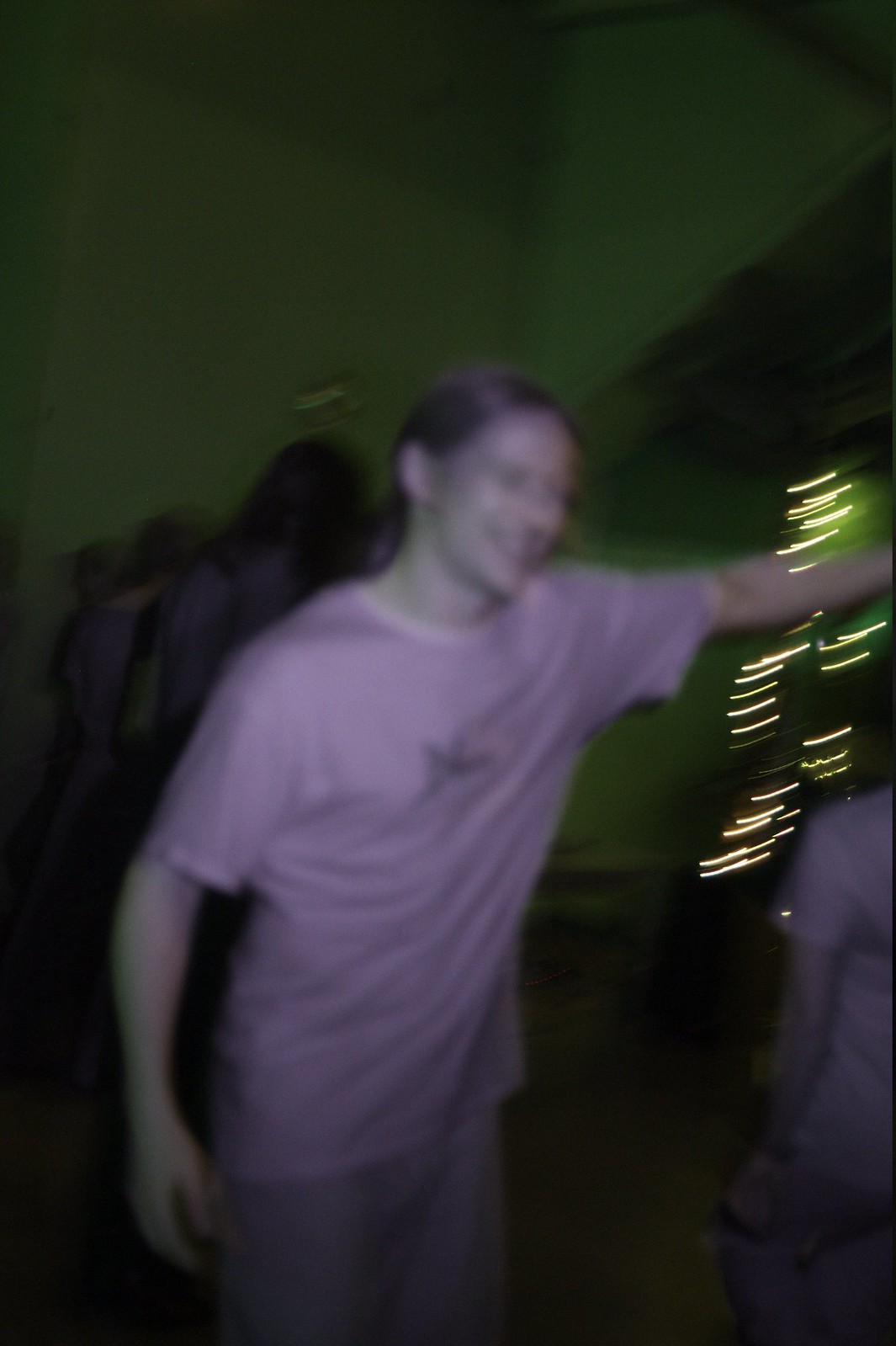The photograph captures a joyful young man, likely in his late teens or early twenties, with shoulder-length hair and a big grin, wearing a pinkish-purple t-shirt. The image appears to have been taken in a dimly lit room at night, creating a somewhat dark and blurry composition. His left arm is raised horizontally, while his right arm hangs down naturally. Despite the photo’s lack of focus, the green lighting that glows on the walls adds an atmospheric backdrop, suggesting a lively setting, possibly a party. Behind him, blurred figures and scattered lights further indicate a bustling environment. To the right, part of another person’s left arm and the back of their shirt are faintly visible. The flash from the camera highlights the young man as the focal point, emphasizing his cheerful demeanor amidst the otherwise indistinct background.